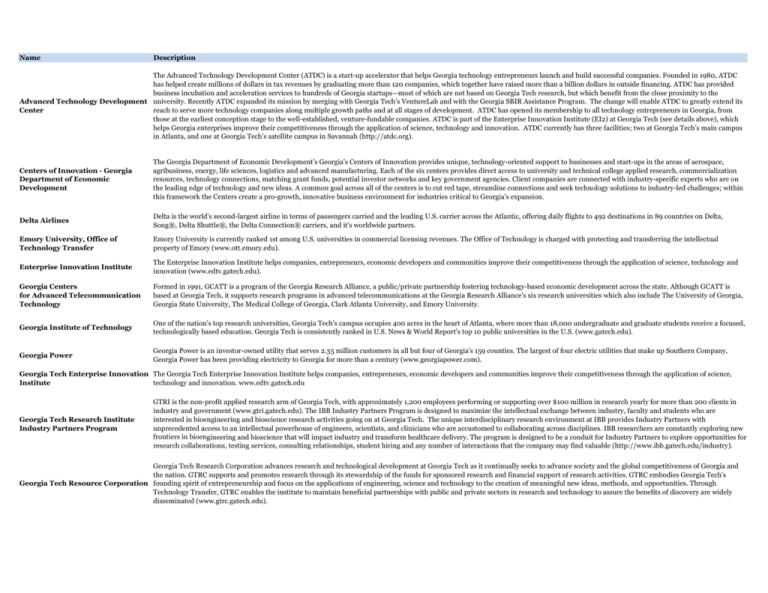This screenshot, likely taken on a laptop, captures a webpage that predominantly features text. The content is set against a clean white background with black lettering, offering high readability. Spanning the top of the page is a distinctive blue banner that features the headings "Name" and "Description" in black text. Below these headings, the page lists various institutions, including the Advanced Technology Development Center, Creators of Innovation, Georgia Department of Economic Development, Enterprise Innovation Institute, Georgia Centers for Advanced Telecommunication Technology, Georgia Institute of Technology, Georgia Power, Georgia Tech Enterprise Innovation Institute, Georgia Tech Research Institute, and Georgia Tech Resource Corporation. The detailed and organized presentation suggests a directory or informational resource pertaining to innovation and technological development in Georgia.